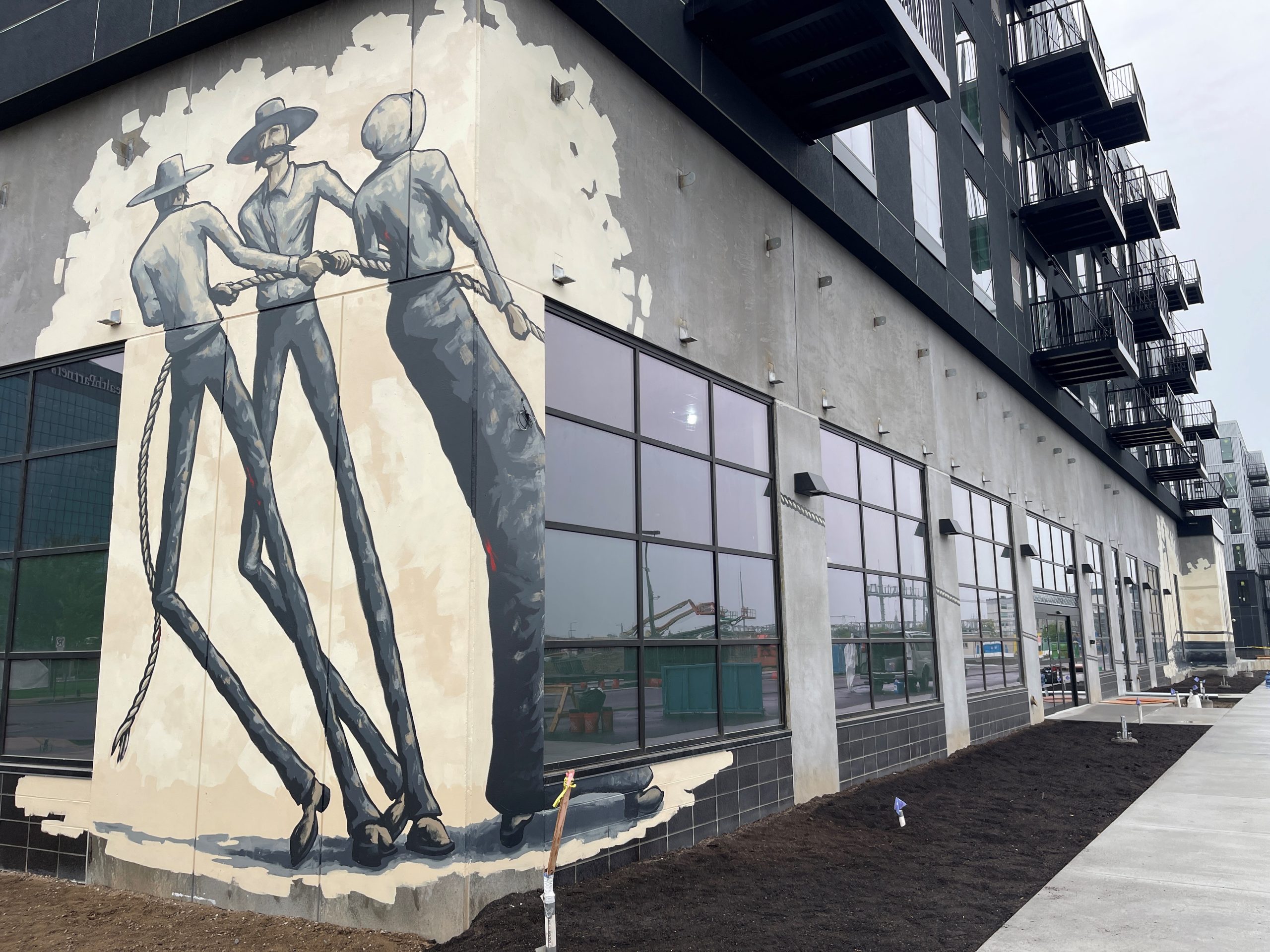The image depicts the corner of a multi-story building, likely four or five stories tall, which appears to be under construction. The building features a combination of black and gray concrete exterior walls adorned with numerous windows. The industrial theme is further emphasized by the inclusion of metal balconies visible on the upper levels. 

On the ground floor, large glass pane windows can be seen amidst the gray concrete facade. Through these windows, construction activity is visible, including cranes and various materials. The ground around the building is currently bare, covered with dirt and mulch, suggesting preparation for landscaping.

Dominating the left corner of the building, there is a striking mural of three tall men with unusually long legs and top hats, dressed in blue shirts and black slacks. They are depicted pulling a rope, adding a touch of artistic flair to the construction site. The image was captured during the daytime, highlighting the ongoing development and the raw, unfinished state of the surroundings.